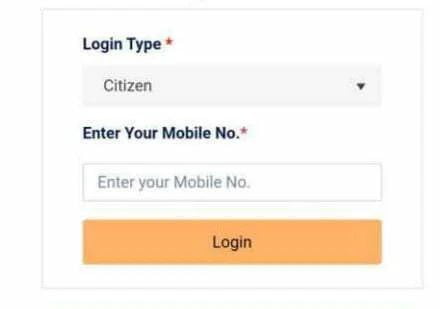This image depicts a section of a website, designed within a clean, white, square frame. The top left, bottom, and right sides of the square are defined by a grey border. Inside the white background, at the top, bold black text labeled "Logon Type" is displayed, with both 'L' and 'T' capitalized. A red asterisk is placed next to the letter 'e' in 'Type'.

Below this, in a grey banner, a dropdown menu shows the option "Citizen" in capitalized black text. Further down the page, the directive "Enter Your Mobile No." is presented in dark print, with 'Enter', 'Your', 'Mobile', and 'No.' capitalized, and accompanied by a red asterisk. This notation indicates a mandatory field for entering a mobile number.

A blank space is provided for users to input their mobile number. Beneath this field, a prominently thicker yellow-orange tab stands out, centrally featuring the word "Login" in black print, with a capital 'L'. This design highlights a call to action for users to proceed with logging into the website.